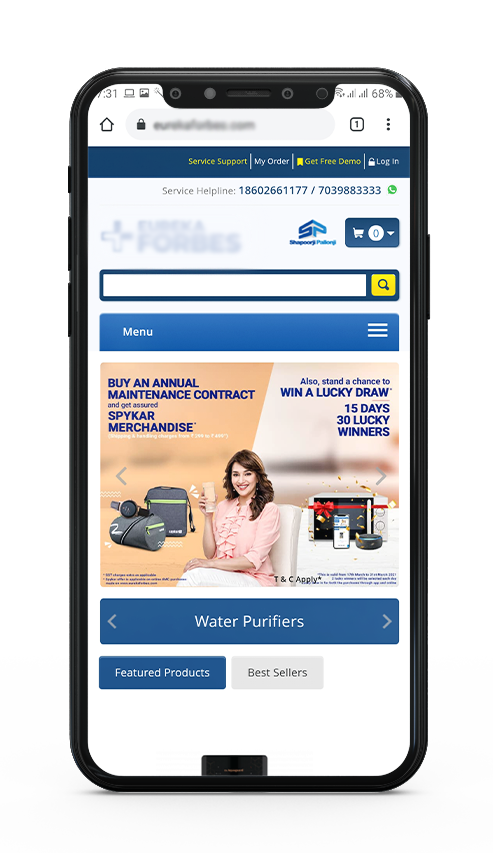The image showcases an entire cell phone with a blurred-out URL at the top. The screen prominently displays the text "Service Helpline" accompanied by contact numbers. Partially obscured text includes the name "Forbes" and a logo resembling a plus sign. To the right, there is a network diagram resembling a tree, alongside a blue shop button. Additionally, there is a search bar with a gold magnifying glass icon and a menu represented by a hamburger icon. 

Below this navigation area, promotional text encourages users to "Buy an annual maintenance contract and get insured spy care merchandise." A woman in a peach-colored top and white pants relaxes with a fancy drink, smiling, and showcasing her auburn hair. Beside her, promotional text announces a "Lucky Draw" with 15 days and 30 lucky winners, with a range of prizes like tablets, laptops, and cell phones.

Immediately under this section, the image highlights water purifiers as the featured product in the "Best Sellers" section. The woman might even be enjoying purified water, aligning with the product focus.